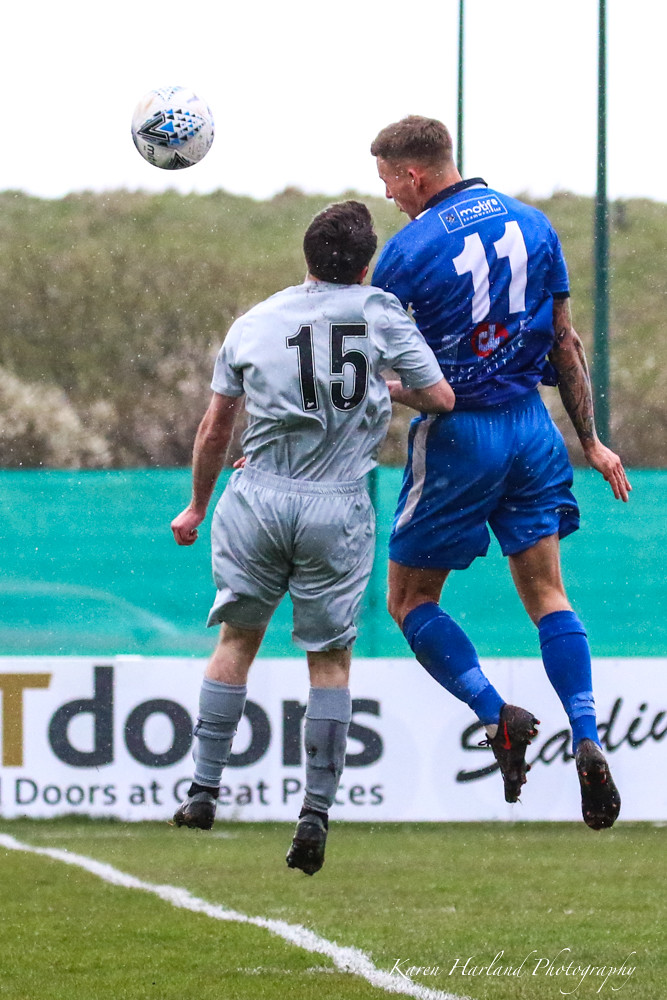This photograph captures a dynamic moment during a soccer game, featuring two players in mid-air as they vie for the ball. The player on the right, dressed in a royal blue uniform with a white number 11 on his back, appears to be leaping higher than his opponent. The player on the left, wearing a gray-silver jersey with a black number 15, has dark brown hair and has jumped to a lower height, with his head reaching about the shoulder level of the player in blue. The soccer ball is suspended in the air above and to the left of the players, suggesting it is either in the process of being headed or is being targeted for a header. The scene is set on a lush green field without visible spectators, bordered by what appears to be another field and a banner that reads "Doors at Great Prices Stadium." The bottom right corner of the image is marked with the inscription "Karen Hartland Harland Photography."